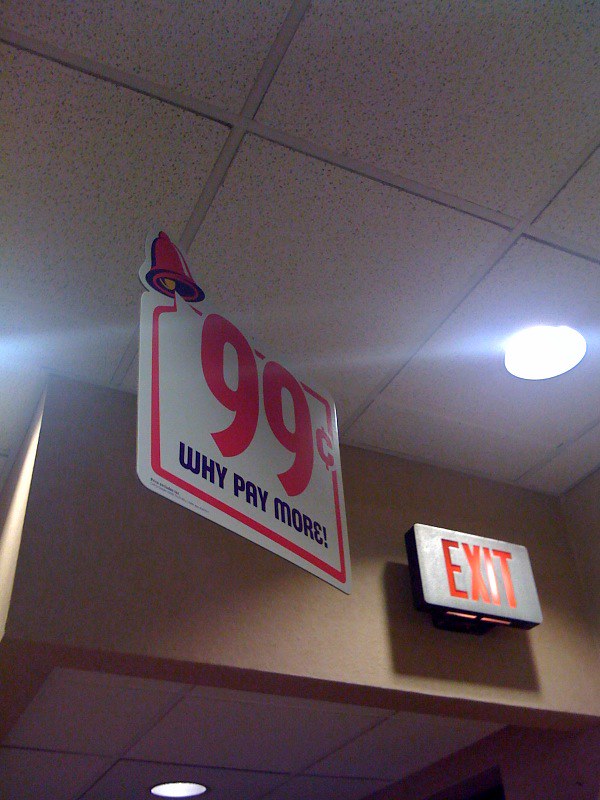In this vertically-oriented photograph, we are looking up at a typical drop ceiling characterized by white tiles peppered with small dots, held up by intersecting aluminum strips. The image prominently captures the ceiling with a touch of beige-colored wall that potentially separates a hallway from another room. Near the top center of the image, a white sign with bold red text reads, "99 cents, why pay more." To its right, affixed to a silver rectangular plaque, the word "EXIT" is displayed in red print. Just in front of the "EXIT" sign, a single recessed light is embedded within the ceiling.